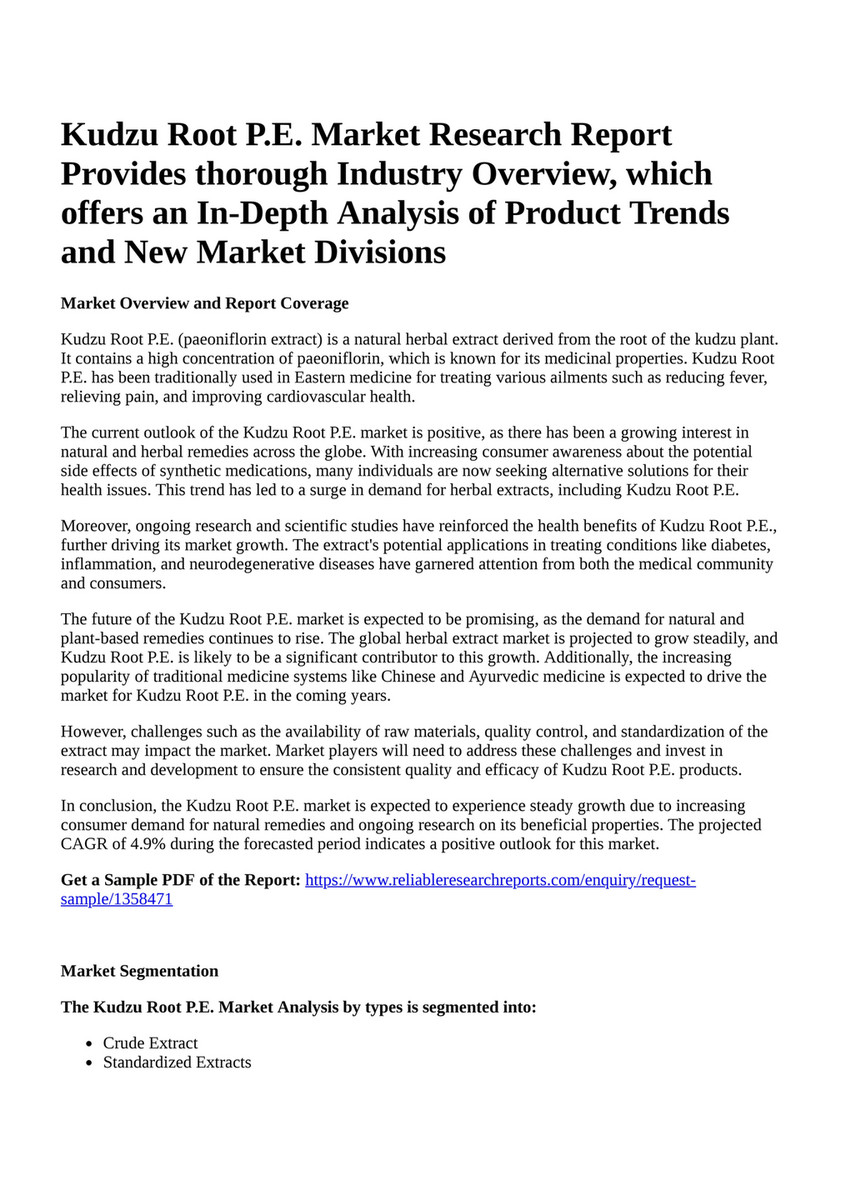The photograph depicts a black and white text document titled "Kudzu Root P.E. Market Research Report Provides Thorough Industry Overview," which offers an in-depth analysis of product trends and new market divisions. Directly beneath the heading are the names of two different authors. Following this are six lengthy paragraphs of extremely small print, described as the "Market Overview and Report Coverage." At the bottom, there is a slightly larger text stating "Get a sample PDF of the report," accompanied by an unreadable blue URL link on the bottom right. Further down, the document mentions "Market Segmentation," detailing that "The Kudzu Root P.E. Market Analysis by Types is segmented into Crude Extract and Standardized Extract" in a bulleted list. This content is formatted in black text on a white background, giving a thorough look at the market analysis.